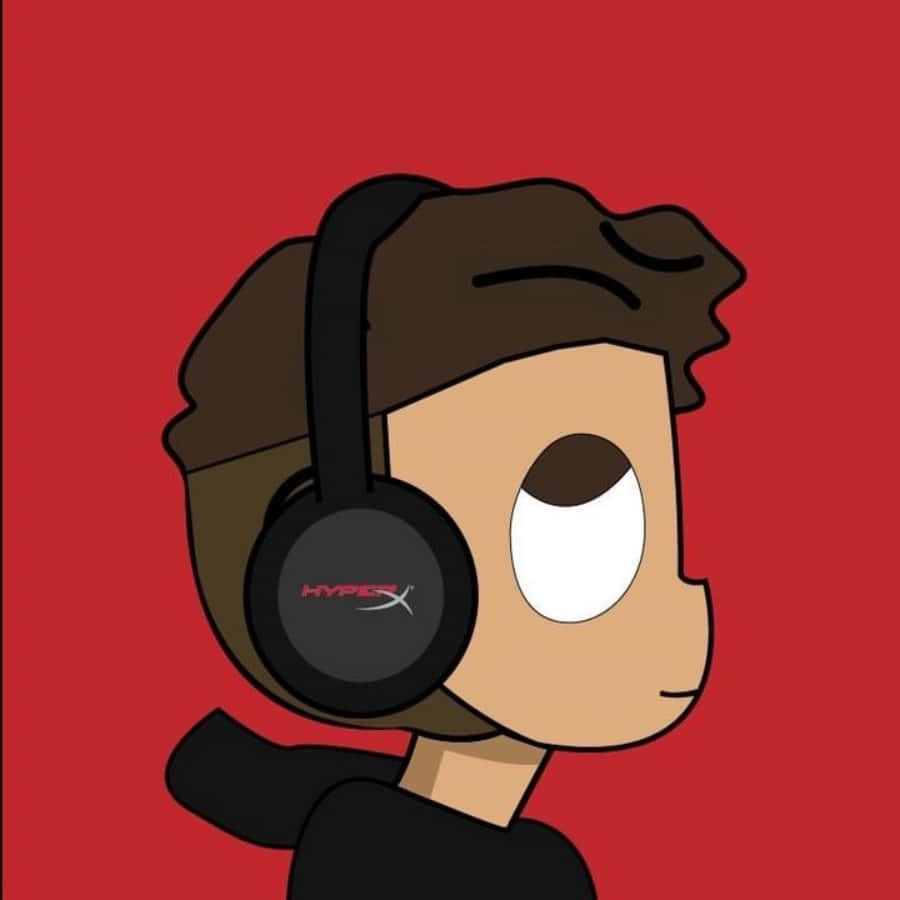The image features a cartoon drawing of a young, light-skinned boy set against a uniform brick-red background. The boy appears to be wearing a black hat or has brown, bushy hair, and sports black headphones with gray circles on the ear cups. Each ear cup has a red "HYPER" written on it alongside a distinctive elongated white "X." He is depicted from the side, showing only his right side profile. His large, brown, egg-shaped eye is looking upwards, with the pupil near the top and the white of the eye at the bottom. His facial features include a small, pointed nose and a simple line for a mouth. He wears a black hoodie, although the hood rests down and is not on his head. The drawing uses shadows to accentuate his neck, giving depth to the cartoon character.